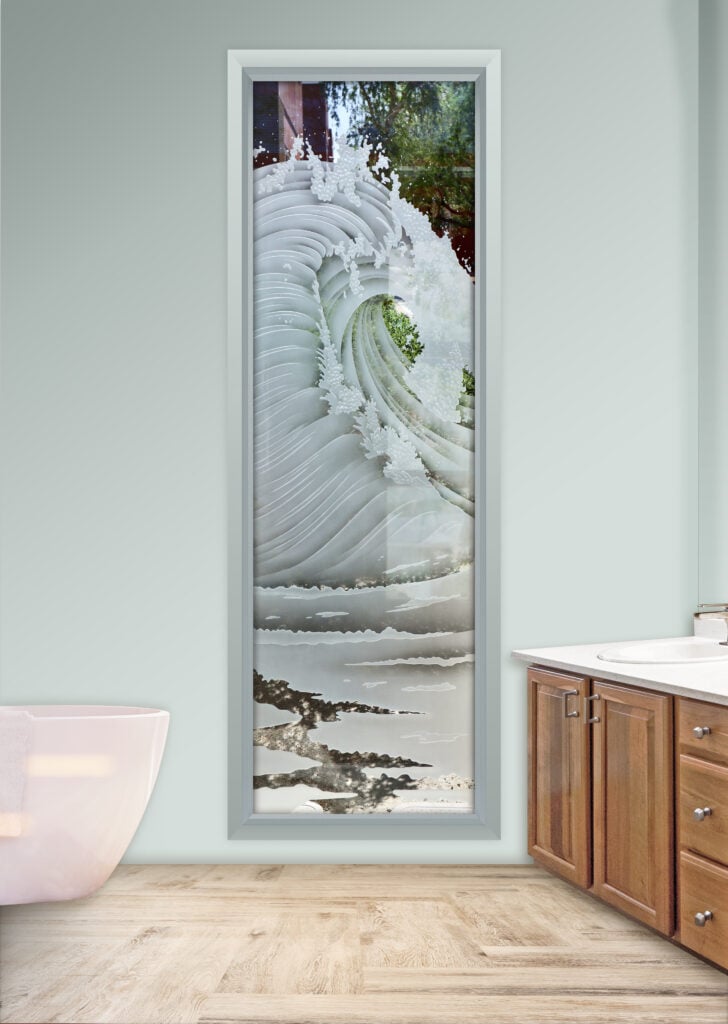The image captures a bathroom with a soothing, light minty green or pale gray-blue wall. Central to the scene is a tall, vertical rectangular painting, possibly about six feet tall and one-and-a-half feet wide, displayed inside a white frame. The artwork showcases a striking depiction of a large white wave rolling in from the right center, curving towards the left center, and descending to the lower right, with touches of brown sand and white water below the wave. In the upper right corner of the painting, there are hints of trees and a wooden post behind the wave.

To the left of the image stands a spacious, white ceramic tub with a towel hanging over its edge. The floor features light brown wood tile, enhancing the bathroom's natural aesthetic. On the right side, there are wooden cabinets and drawers with silver handles and knobs. The cabinetry arrangement includes two doors and three drawers, accompanied by a white marble countertop housing a white sink and an exposed faucet. Overall, the bathroom exudes a serene and harmonious blend of natural elements and modern fixtures.